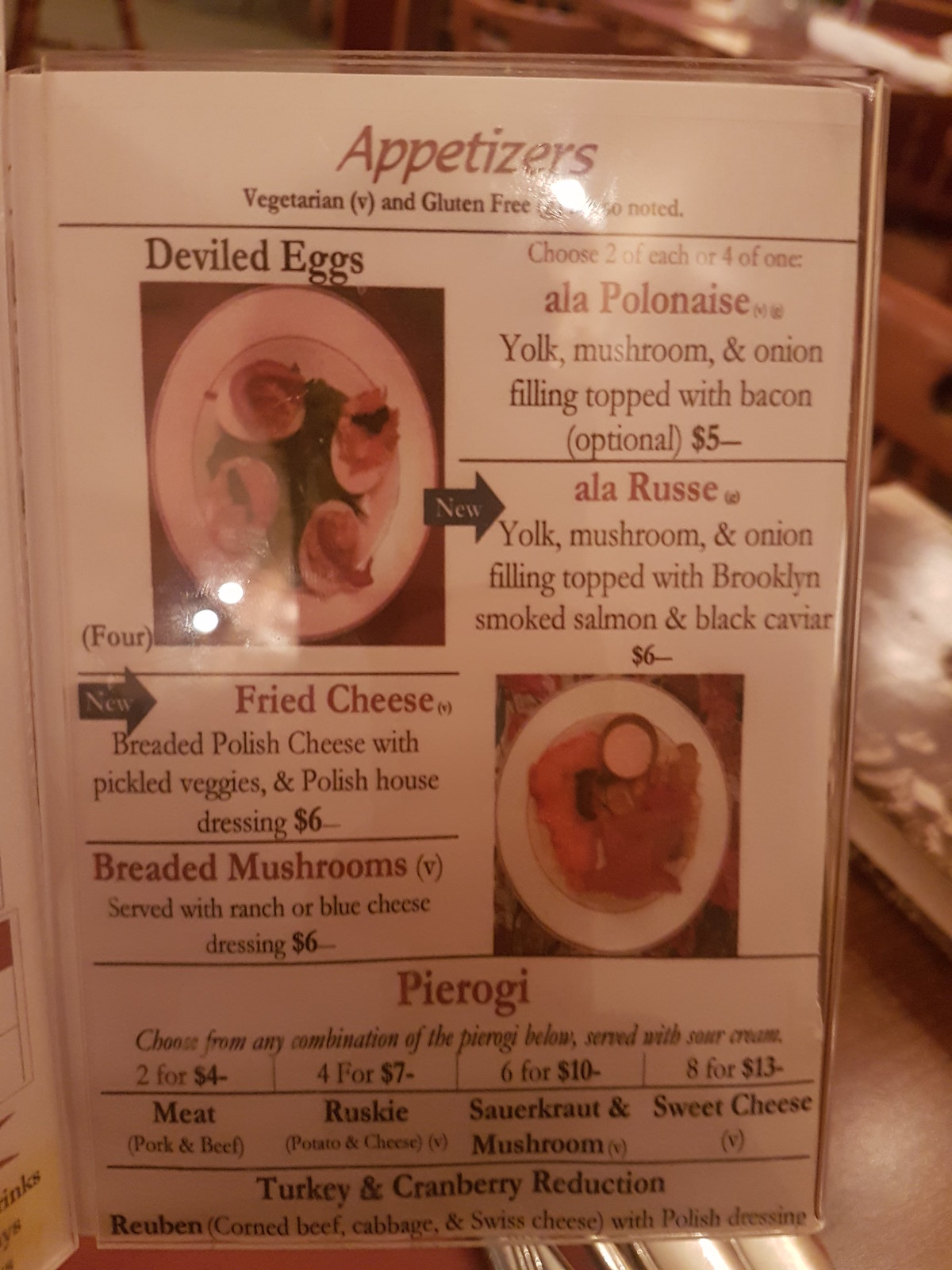A close-up image captures an intimate view of a menu seen through the eyes of someone actively perusing its contents. The menu, standing upright on a dark brown tabletop, reveals the right-hand page of a beige-colored paper. This illuminated page is titled "Appetizers" at the top. 

In the top left corner, a labeled image showcases a plate of deviled eggs. Adjacent to it on the top right, various egg-based entrées are listed. The center of the page prominently features the items "Fried Cheese" and "Breaded Mushrooms" in dark brown lettering. Just to the right of this list, a dark brown silhouette depicts a white plate with an egg and some brown accompaniments.

At the bottom center of the page, the word "Pierogi" is displayed in brown lettering. Below, in fine black print, are the four types of pierogi available: Meat, Rusky, Sauerkraut and Mushroom, and Sweet Cream. The menu's detailed descriptions and visuals suggest a diverse range of appetizer offerings, inviting the reader to explore further.